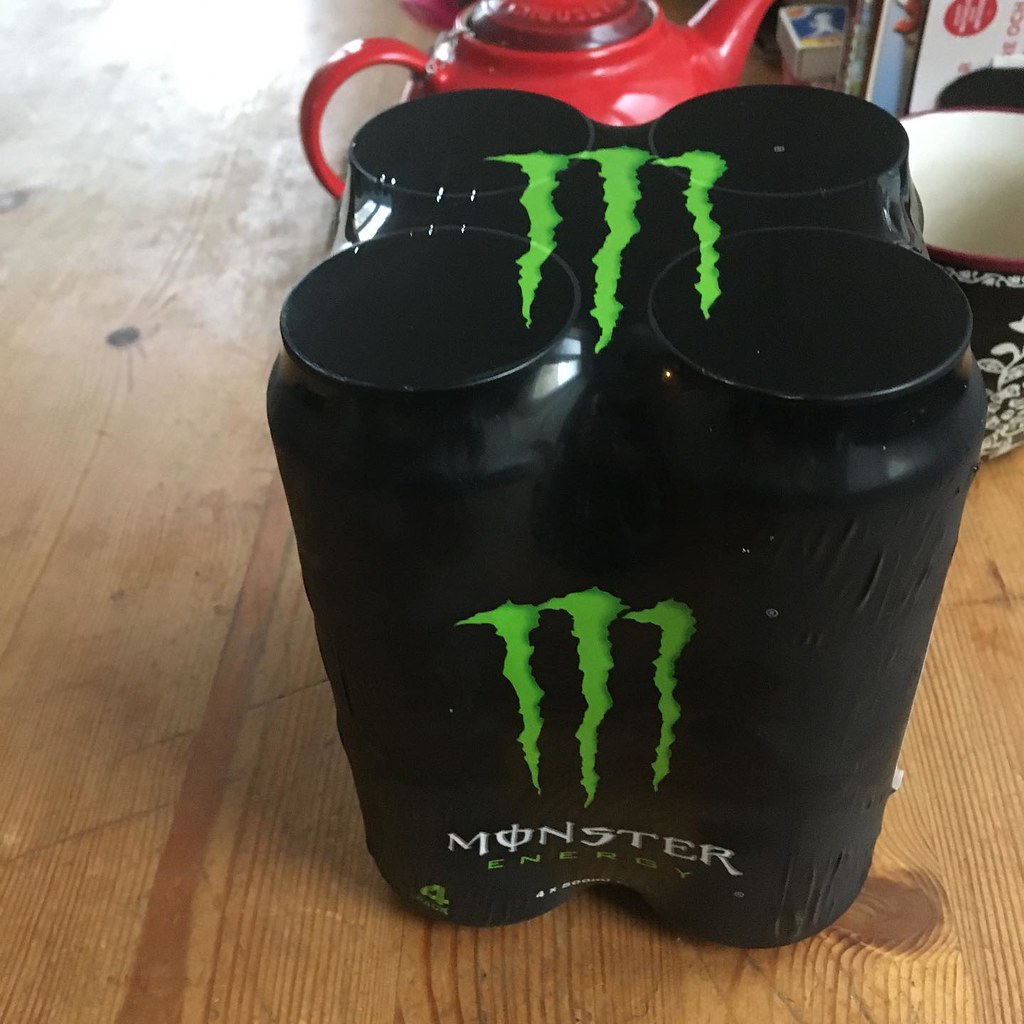The image shows an overhead view of a 4-pack of Monster Energy drinks tightly wrapped in black shrink-wrap packaging. Each can features the iconic neon green "M" logo that resembles claw marks. The packaging also displays the brand name, with "Monster" in white and "Energy" in green. This 4-pack is placed on an older, light wood table with visible grain, illuminated by sunlight from the top left corner. Directly behind the Monster pack is a black coffee mug, with a white interior and adorned with a white floral design. To its right is a ceramic red teapot with a matching lid. Scattered around the table in the background are additional kitchen items such as magazines and matches, adding more context to the setting.